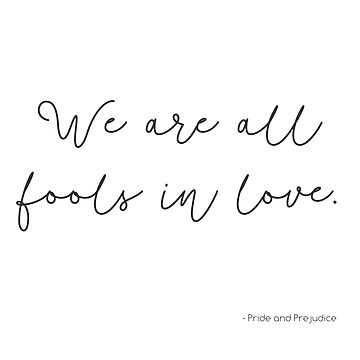The image is a minimalist quote card with a completely white background and a famous quotation from the book "Pride and Prejudice." The main text, written in a modern cursive script, states in black letters: "We are all fools in love." This text is split into two lines with "We are all" on the first line and "fools in love." on the second, concluding with a period. In the bottom right corner, the quote is attributed to "Pride and Prejudice" in a smaller, simpler black font, preceded by a dash. The overall design is clean and uncluttered, highlighting the poignancy of the quote.